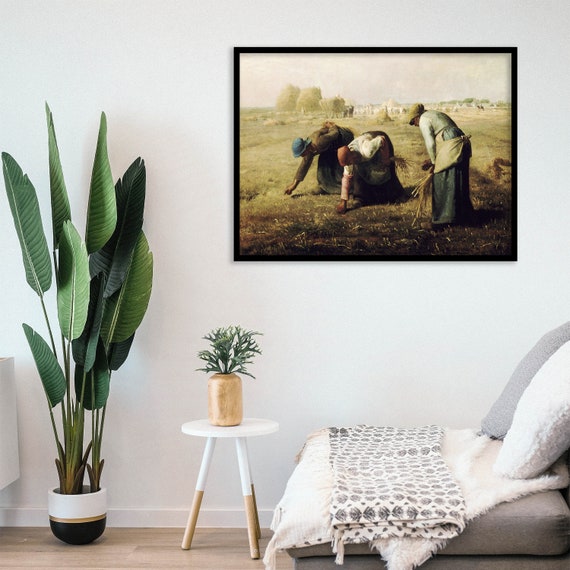The image depicts a cozy interior space within a home. The black wall prominently showcases a framed painting of three women working on a farm, either picking or harvesting plants. Below the artwork sits a grey armless chair adorned with a white and grey pillow on one side and a white cloth with a black pattern draped over it. On the left side, an indoor plant with large, elongated leaves stretches upwards. Positioned between the chair and the plant, a small, round white table with three golden legs supports a smaller pot filled with greenery. The scene combines elements of comfort and natural decor, highlighted by subtle detailing and thoughtful placement.